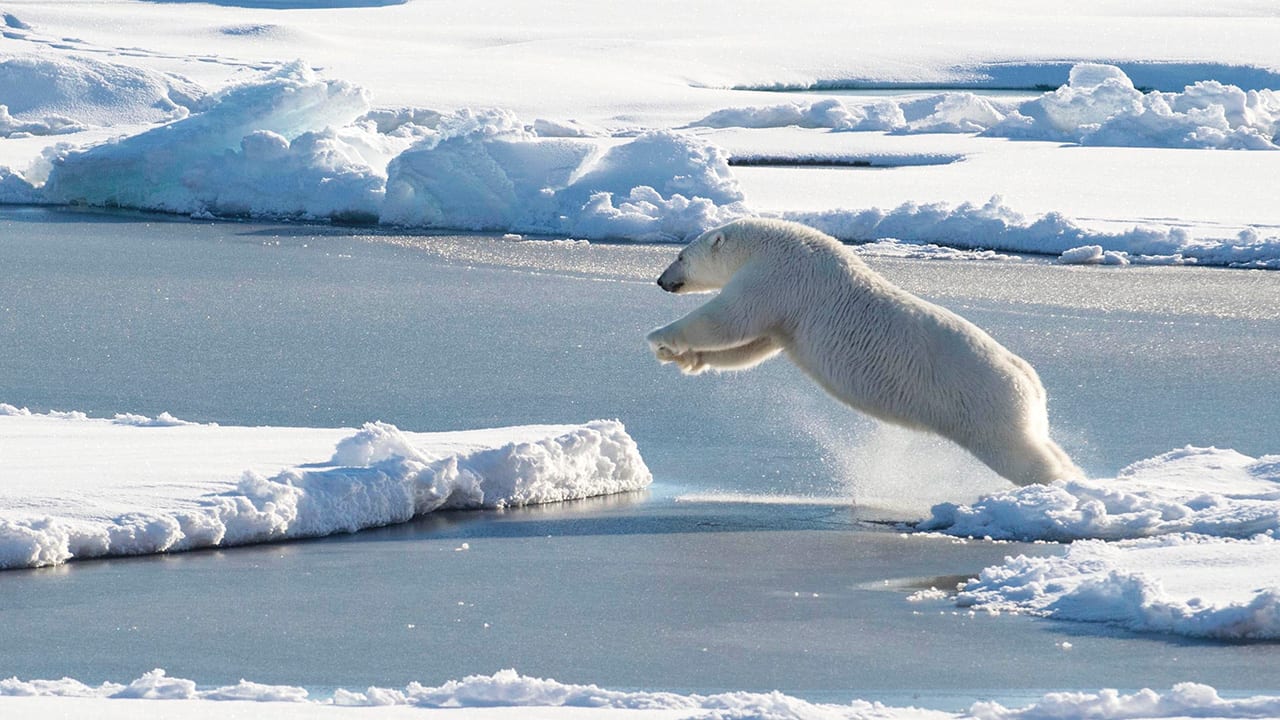In this captivating photograph likely taken in the Arctic, a solitary polar bear is caught mid-jump, leaping from one fragment of ice to another against the backdrop of a frigid, snow-covered landscape. The polar bear, with its white fur contrasting sharply against the blue of the glacial water, is springing off its hind legs with its front paws stretched out ahead, showing a sense of urgency and agility. The water below, dotted with more ice, appears partly frozen, emphasizing the precarious nature of the bear's crossing. This image, reminiscent of classic National Geographic magazines, might evoke thoughts on environmental issues such as global warming, highlighting the bear's struggle to navigate the shrinking icy terrain.